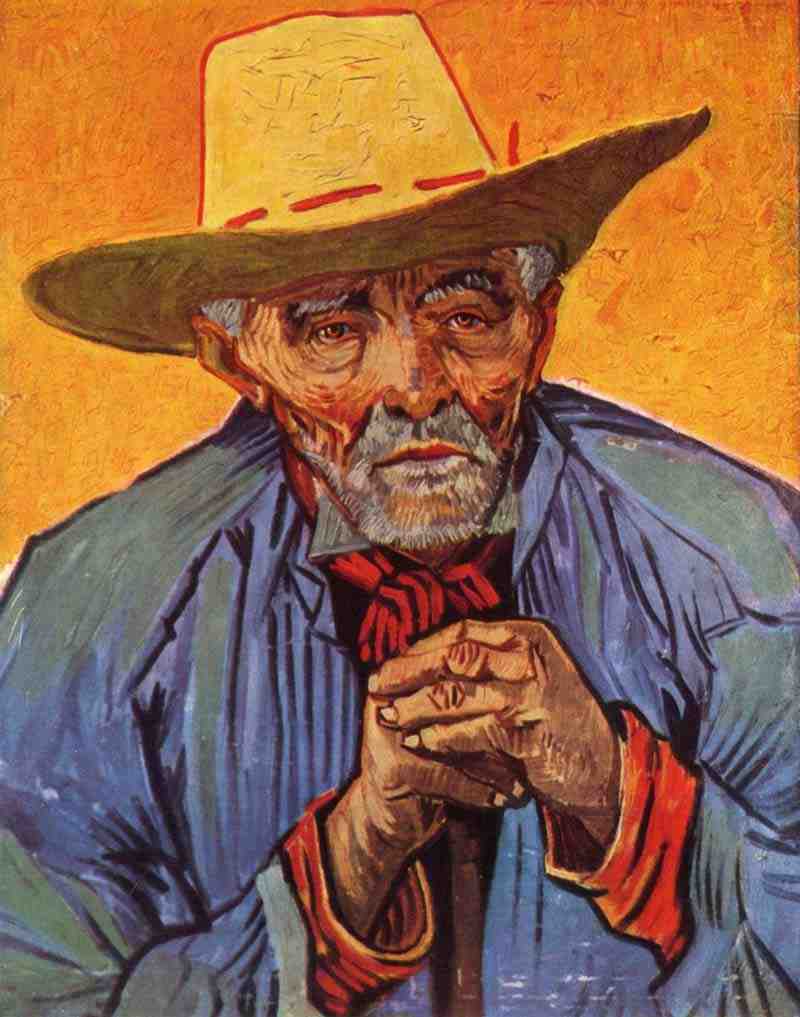The painting depicts an older Hispanic-looking man with dark skin and a gray beard and mustache, set against an orange background. He wears a yellow straw hat with a red string woven through it, and his expressive face is marked with wrinkles, adding character to his aged visage. The man is dressed in a textured blue coat, with shades of green and blue, layered over a red shirt, the cuffs of which peek out from the sleeves of the coat. His attire is further accented by a red tie. He holds a cane in front of his chest, with his right hand positioned under his left, emphasizing the thoughtful pose and the intricate details of his clothing.